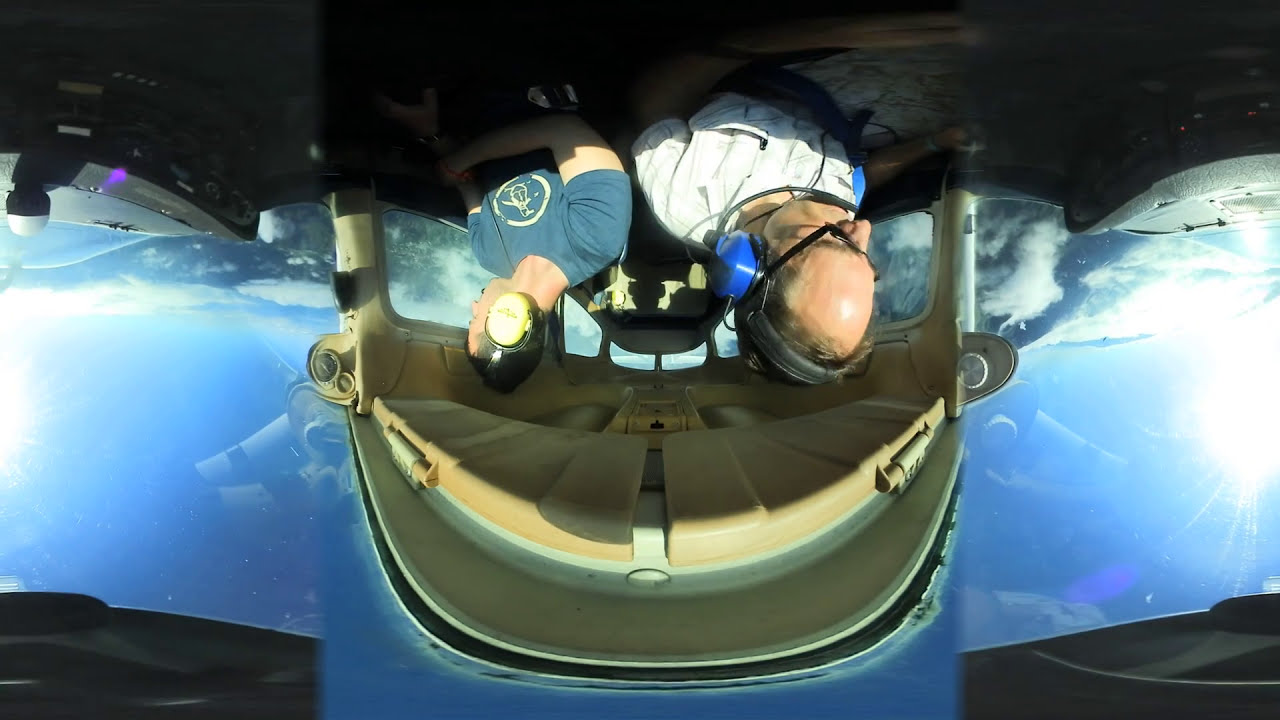This unique outdoor daytime photograph, approximately six inches wide and three inches tall, captures an intriguing moment inside a small, two-person airplane through a fisheye or wide-angle lens, lending a distinctive curved distortion to the image. The photograph is upside down, presenting an unusual perspective. At the center, two Caucasian men are seated next to each other. The man closer to the viewer is older, balding, and wears sunglasses, over-the-ear blue headphones, and a white shirt with stripes. He appears focused, possibly looking at a map. The younger man sitting beside him has black hair, wears similar headphones, and dons a blue t-shirt featuring what looks like a penguin. The airplane's interior roof, adorned in green and orange hues, arches above them. The view out of the airplane's windows displays a bright blue sky dotted with white clouds and sunshine on either side of the men. Despite the daytime setting, a mirror and lights are visible within the plane's console. Hints of a valley, with grass and a cityscape, can be glimpsed below, adding to the photograph's vibrant outdoor atmosphere.